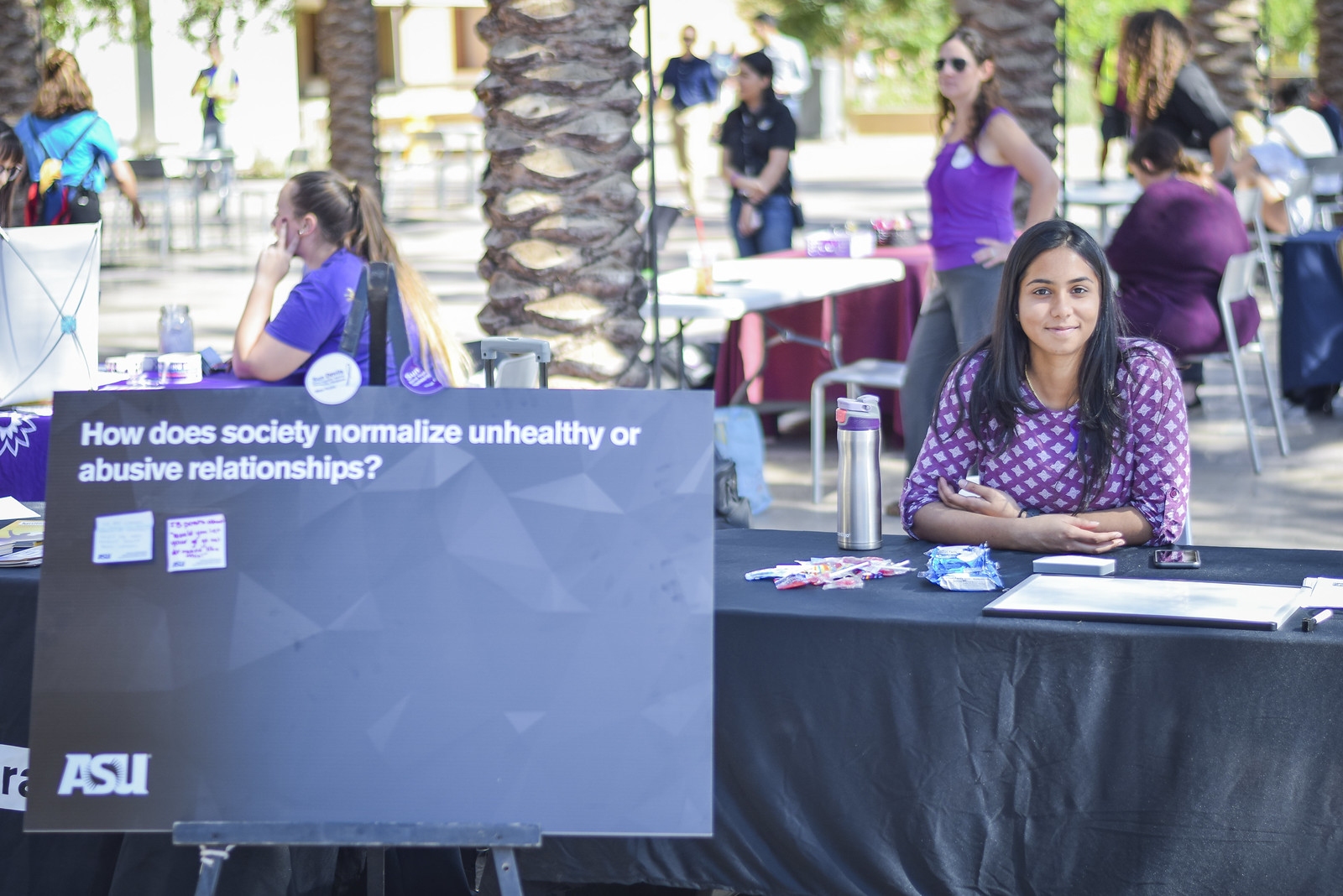The image depicts an outdoor event, likely on a college campus, framed in landscape orientation. Central to the photograph is a young woman, approximately 23 years old, with long dark hair, smiling directly into the camera. She wears a purple and white blouse and sits at a table with a black drape, her arms folded, with various materials in front of her, possibly for distribution. The setting appears to be a fair or informational event, as suggested by the adjacent tables forming an enclosure and the various individuals, both men, and women, milling around in the background. Behind the woman, other participants, also in purple shirts, interact with attendees. A prominent gray sign in the foreground reads, "How Does Society Normalize Unhealthy or Abusive Relationships?" with two white note cards pinned on it and the "ASU" logo in the bottom left corner. The scene is further set by palm trees visible between the tables, enhancing the outdoor campus atmosphere.